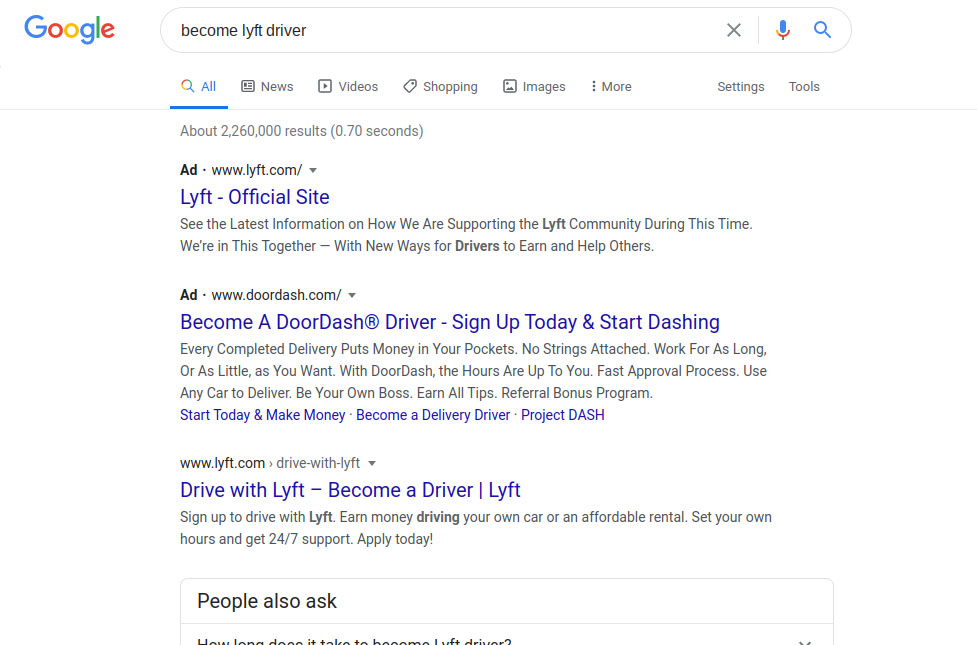Google Search Results for "Become Lyft Driver"

This image displays a screenshot of Google search results with a clean, white background. At the top-left corner is the multicolored Google logo. To the right of the logo is the search bar, which has a thin, light-gray outline. The query "Become Lyft Driver" is typed in black text on the left side of the search bar. Adjacent to the typed text, on the right side of the search bar, there's a light-gray 'X' icon followed by a thin, light-gray vertical separator line. Further to the right, there is a multicolored microphone icon and a blue magnifying glass icon.

Below the search bar, a series of navigational tabs are displayed, each accompanied by an icon and label. The first tab, positioned just below the search bar on the left, is marked with a multicolored magnifying glass icon and the word "All" in blue text, underneath which is a blue underline indicating it's the active tab. The subsequent tabs, displayed in medium gray, are:

- "News" with a newspaper icon
- "Videos" with a square containing a right-pointing triangle icon
- "Shopping" with a shopping tag icon
- "Images" with a picture icon
- "More" with three vertically stacked dots icon

To the far right, following some negative space, there are "Settings" and "Tools" options.

A thin gray line runs horizontally underneath this navigation bar, aligned with the blue underline of the "All" tab. Below this line, light-gray text indicates, "About 2,260,000 results (0.70 seconds)."

The search results appear below this indicator, each entry consisting of blue titles with medium-gray descriptions. The first result on the top left starts with bold black text reading "Ad," followed by a gray dot, "www.lyft.com/" and a gray downward arrow. The blue text link titled "Lyft - Official Site" appears below, followed by two lines of description, with succeeding results following a similar layout.